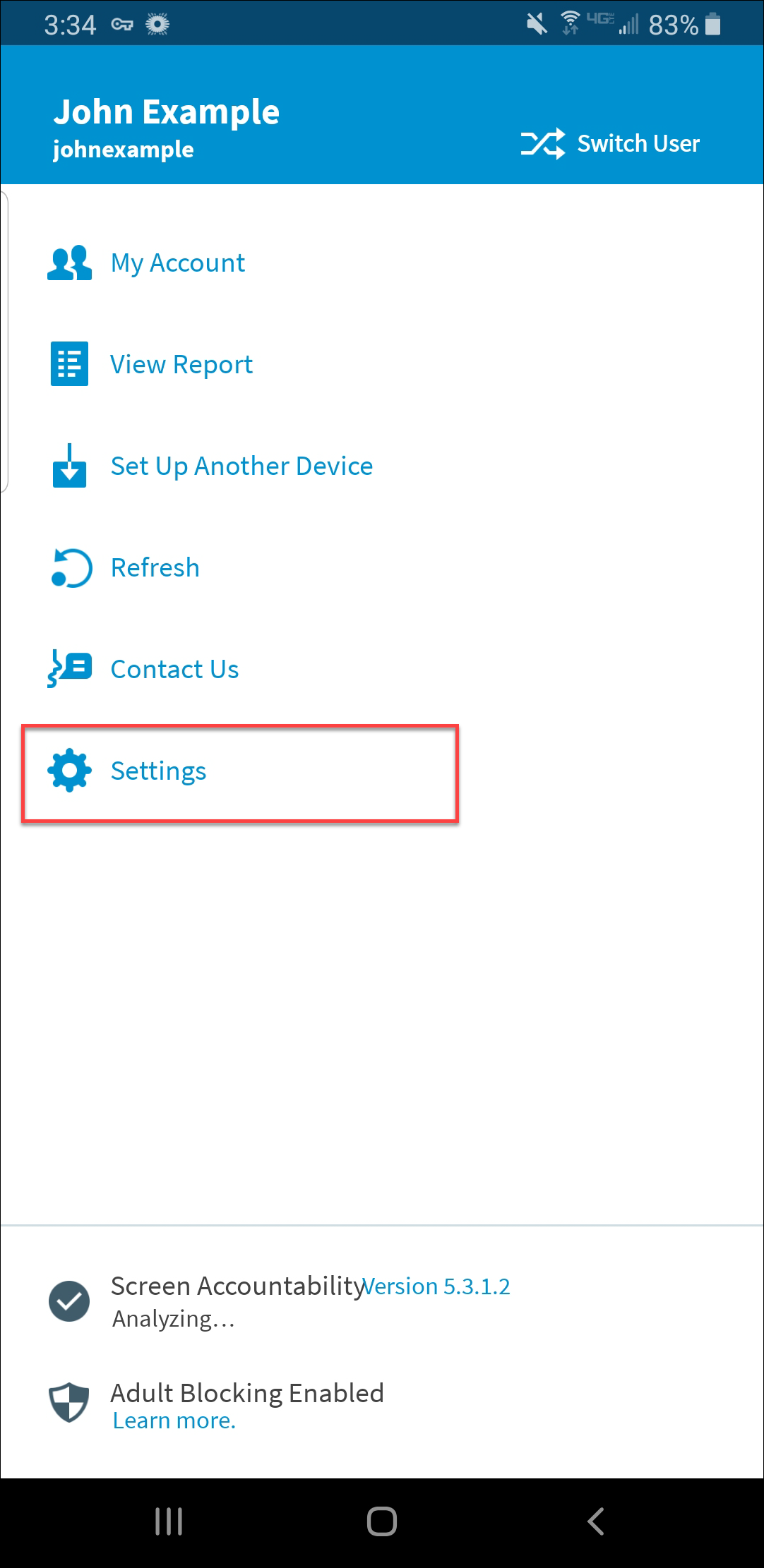In this image, there is a screenshot of a mobile device displaying detailed status information and options. 

At the top left corner of the screen, the current time is shown as 3:34. Adjacent to the time, the VPN logo is visible in the status bar. Moving to the top right of the screen, we observe the mute icon indicating that the device is on silent mode. The Wi-Fi signal strength is at its maximum with 4 out of 4 bars, while the 4G LTE signal is weaker and is displaying 2 out of 5 bars. The battery level is also visible, showing a charge percentage of 83%.

Below the status bar, there is a list of options and informational text:
- "John Example" (possibly indicating the current user)
- "Switch User"
- "My Account"
- "View Report"
- "Set Up Another Device"
- "Refresh"
- "Contact Us"
- "Settings"
- "Screen Accountability Version 5.3.1.2"
- "Adults Blogging Enabled"
- "Learn More"

This comprehensive screenshot displays essential device status indicators along with various user options and settings related to account management and device setup.